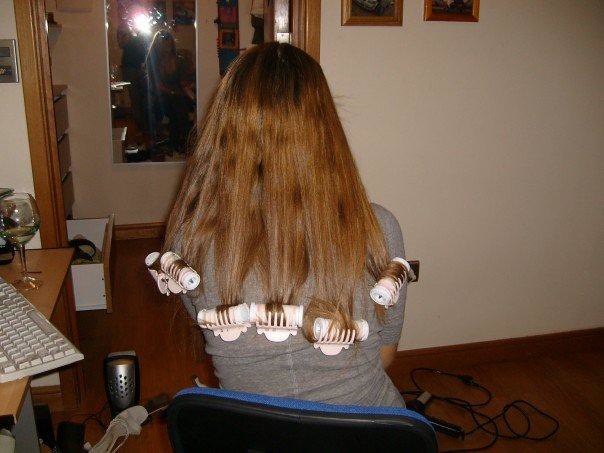In this detailed photograph, we see the back of a girl seated in a chair on a dark brown wooden floor. She is wearing a gray shirt with sleeves reaching her elbows. Her long, reddish-brown hair extends to the middle of her back and is partially styled with white plastic curlers. Specifically, about six curlers are positioned at the tips of her hair, aiming to create a wavy or curly effect. The chair she sits on has a black backrest with a blue cushion. 

The background includes a white wall adorned with a couple of indistinct picture frames. To the left, there is a desk that holds an old-style gray keyboard and a wine glass containing some white wine. Beneath the desk is an open drawer, though its contents are unclear. A mirror situated in the distance reflects a partial, indistinct image of the front of the girl and the person taking the photo, enhanced by the camera's flash. Additionally, a brown baseboard lines the bottom of the wall, and an open closet space can be seen on the left-hand side, further enriching the room's setting.